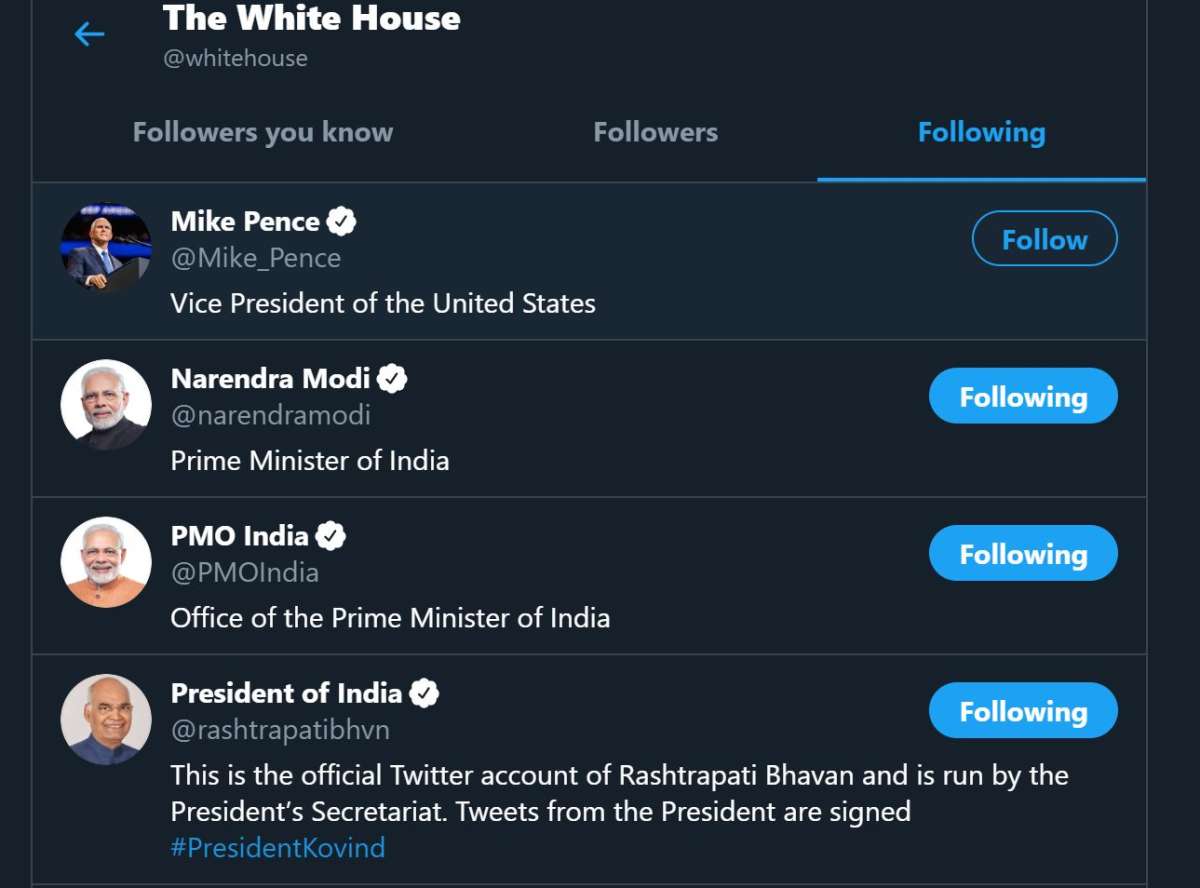The image depicts the Twitter profile page of the White House, characterized by a black background theme. The interface displays sections such as 'Followers you know', 'Followers', and 'Following'. In the 'Following' section, notable accounts are listed. One highlighted user is Mike Pence, indicated by a white tag beside his name. Additionally, the profile of Narendra Modi appears, verified with the blue checkmark badge. His profile description reads, "Prime Minister of India, @PMOIndia," and points to the official Office of the Prime Minister of India. The text also mentions the President of India at Rashtrapati Bhavan. The detailed layout showcases the prominent figures the White House account is connected with.